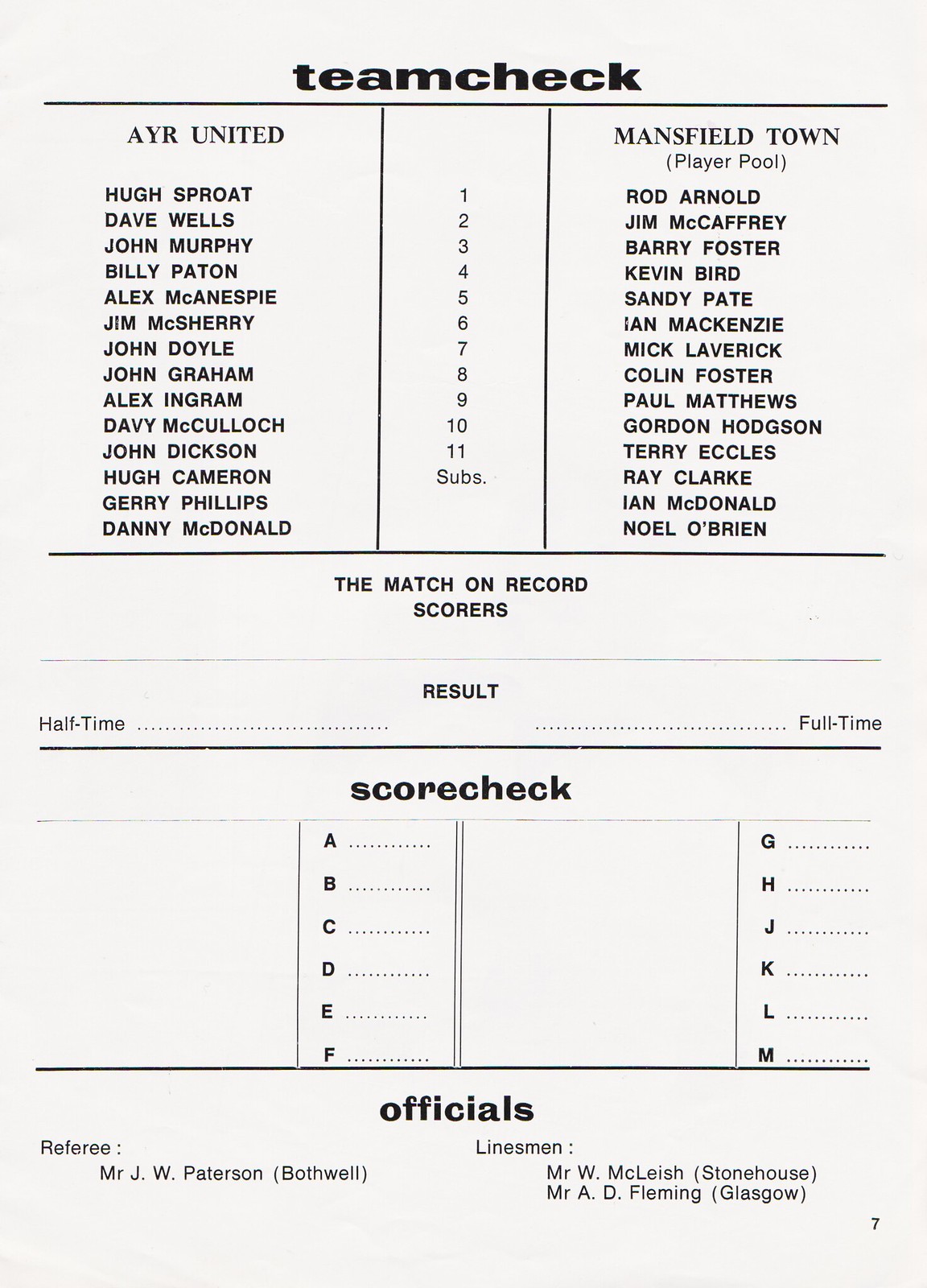This image depicts page seven of a vintage sports magazine, presumably dedicated to a soccer or football club program. The page is in portrait orientation, featuring black text on an off-white background. At the very top, "Team Check" is boldly printed, setting the thematic tone of the page. Below this heading are three distinct columns. The left column is titled "AYR United" and lists the names of 11 players along with three substitutes. The center column is narrow, simply numbered 1 through 11 with "Subs" listed underneath. The right column is labeled "Mansfield Town (Player Pool)," also detailing 11 players and three substitutes, aligning the names neatly on the left-hand side. 

Beneath these columns, a horizontal section is titled "The Match on Record Scorers," though it leaves spaces for the scores to be filled in manually. Further down, another area labeled "Score Check" is divided into two vertical columns—letters A through F on the left, and G through M on the right, with blank lines beside each letter for score entries. At the very bottom, the word "Officials" is prominently displayed, listing the referee and linesmen's names. This page, characterized by its structured layout and concise content, captures the essence of a vintage print publication dedicated to documenting team rosters and match details.